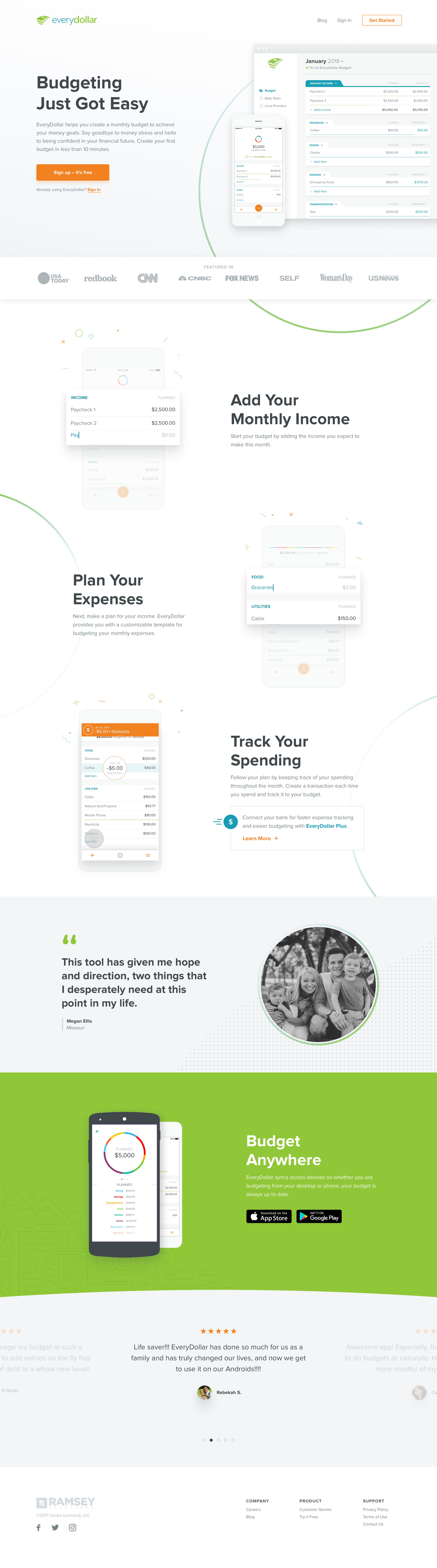A screenshot of a website promoting easy budgeting features is displayed. The header prominently states, "Budgeting Just Got Easy," with small print details beneath it. Below this is an eye-catching orange bar, all contained within a light gray box. To the right of this section is a visually highlighted chart in light green. 

Underneath the chart, a white horizontal line divides the content, leading to another chart labeled "Add Your Money." Further down, the text "Plan Your Expenses" is accompanied by an indistinct circular graphic. To the right of this is another circular image.

The page features images of spreadsheets, though one is too small to make out clearly. The text "Track Your Spending" appears, alongside a brief guide on how to manage finances. Below this, a separate section begins with a gray top, a distinctive lime pink middle, and a gray bottom. An icon depicting a woman accompanied by others, rendered in black and white, appears next to another bit of explanatory text.

Finally, there's an image of an iPad towards the bottom of the screenshot, adjacent to further information presented on a gray background.